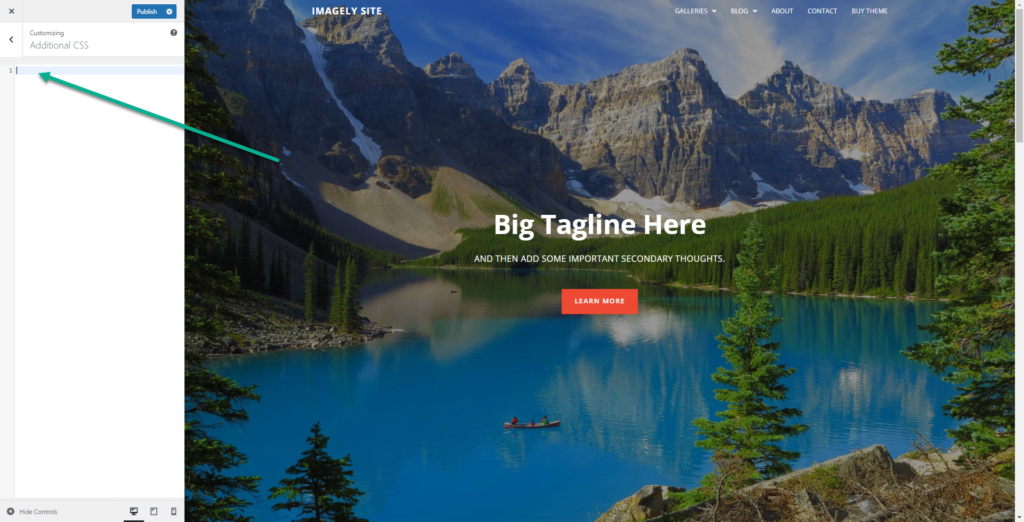The web page features a stunning background depicting a serene landscape. Dominating the scene are majestic, rocky mountain peaks rendered in varying shades of grey and deep dark brown. At the base of these mountains, a dense forest of tall pine trees stretches out, meeting the shoreline of a tranquil, blue lake. The lake spans the lower portion of the image horizontally, mirroring the rugged mountains in its calm waters. A small boat floats on the lake, with the outlines of three people seated inside it. Across the forefront of the image, large white text proclaims, "BIG TAGLINE HERE," adding a striking textual element to the picturesque vista.